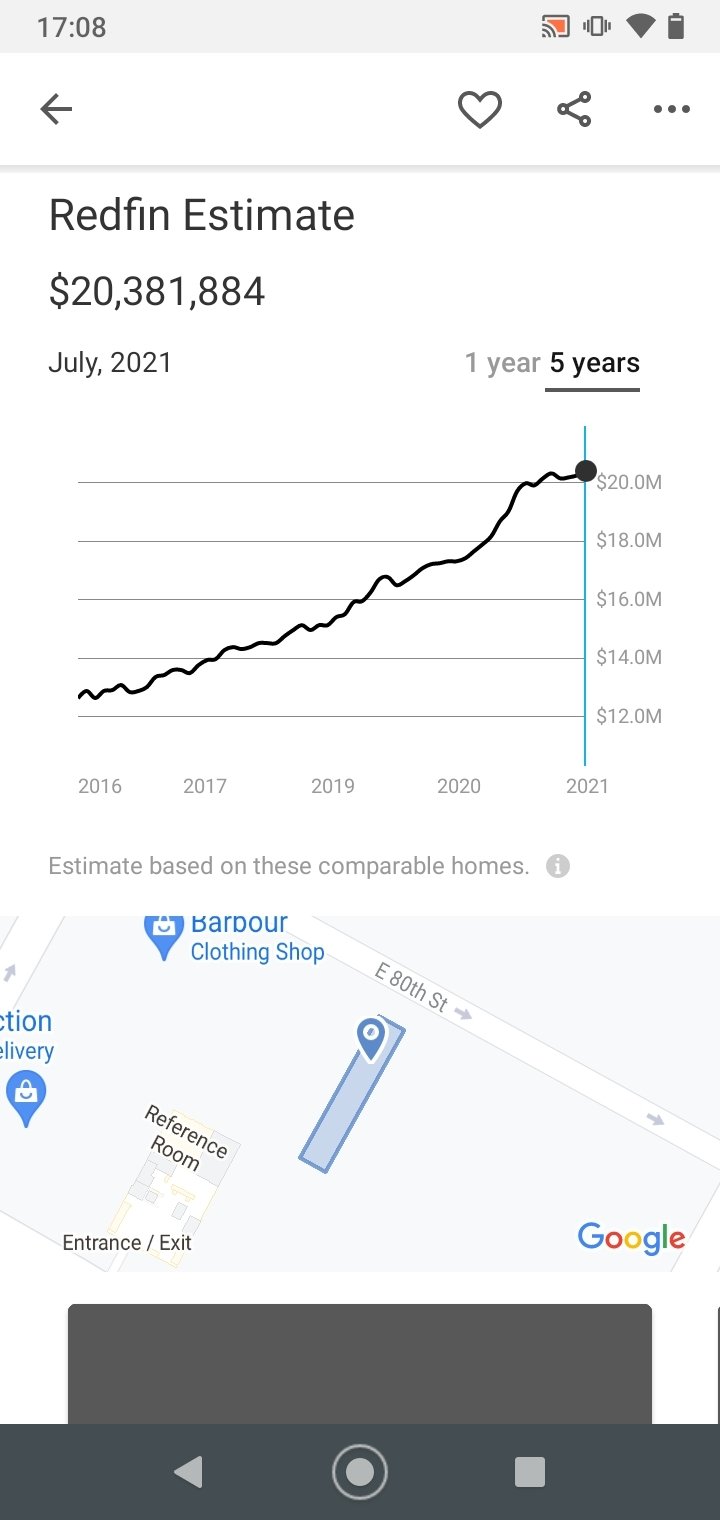This detailed caption describes the image captured on a cell phone screen:

"The photo shows a Black and White Redfin Estimate graph, as viewed on a cell phone. The graph, which resembles a bar or line graph, documents property estimates over a span of five years—specifically 2016, 2017, 2019, 2020, and 2021. The title 'Redfin Estimate' is clearly visible at the top of the graph, with a highlighted figure of $20,381,884 labeled under July 2021. The graph itself begins at $12 million on the vertical axis and ascends in increments of $2 million, reaching up to $20 million. Notably, a black line traces this value progression over the years marked on the horizontal axis at the bottom.

Beneath the graph, a small map is visible with various businesses labeled, including a barber shop and a clothing store, among other locations. The map adds context to the geographical area relevant to the estimate value displayed above."